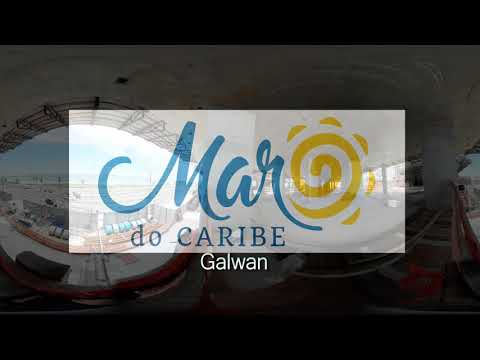This image depicts a transparent logo centered on an outdoor panoramic scene. The background shows a distant open area, possibly a beach or an open parking lot, under a partly cloudy sky with visible tables, water, and some scaffolding at the top. The logo itself is enclosed in a solid transparent white rectangular horizontal box. At the center of the box, the word "MAR," is written in blue cursive letters, with a yellow swirl resembling the sun integrated into the script. Beneath "MAR," the words "do CARIBE" are inscribed in blue. Further below, the word "Galwan," spelled G-A-L-W-A-N, is featured. The image has a dark overlay, contributing to an advertisement-like style and is framed by a black border at the top and bottom. The scene captures a blend of daytime outdoor colors, including shades of blue, white, yellow, red, tan, and orange, providing a vivid and detailed backdrop for the logo.